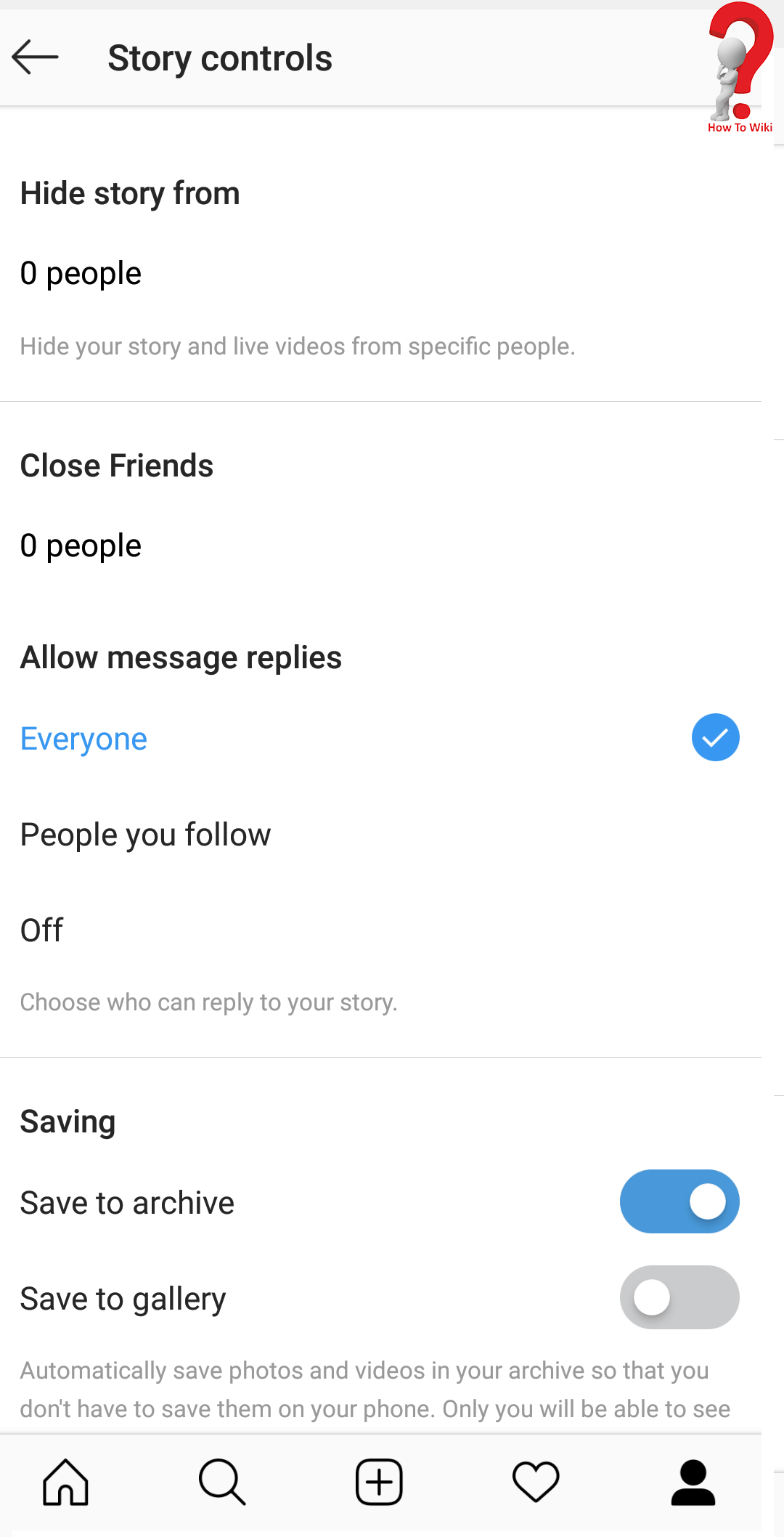This image is a screenshot of a settings page from a mobile application. The interface is designed with a light gray header at the top, featuring a black arrow pointing to the left, followed by bold text reading "Story Controls." On the far right of this header, there is a three-dimensional white stick figure leaning against a red, three-dimensional question mark with the label "HowToWiki" in red text underneath.

The main body of the settings page has a white background and is organized into sections separated by thin gray lines. The first section is labeled "Hide Story From" in bold text. Below this heading, it reads "Zero People" in black text, and beneath that, a brief description in small gray text says, "Hide Your Story and Live Videos from Specific People."

The second section is titled "Close Friends," followed by "Zero People." It continues with the option "Allow Message Replies" marked with "Everyone" in blue text, accompanied by a blue circle with a white check inside it, indicating selection. Below this, it says "People You Follow" set to "Off," with small gray text underneath that reads, "Choose Who Can Reply to Your Story."

The third section is focused on "Saving" options. It includes "Save to Archive" with a blue pill button indicating it is turned on (the white circle is on the right). Below this, the "Save to Gallery" option shows a gray pill button with the white circle on the left, indicating it is turned off. This section is accompanied by small gray text that explains, "Automatically Save Photos and Videos in Your Archive so that you don't have to save them on your phone. Only you will be able to see it."

At the bottom of the page, there is a light gray footer containing several icons: from left to right, there is a house icon, a magnifying glass, a plus sign inside a box, a heart, and finally, a black icon of a person.